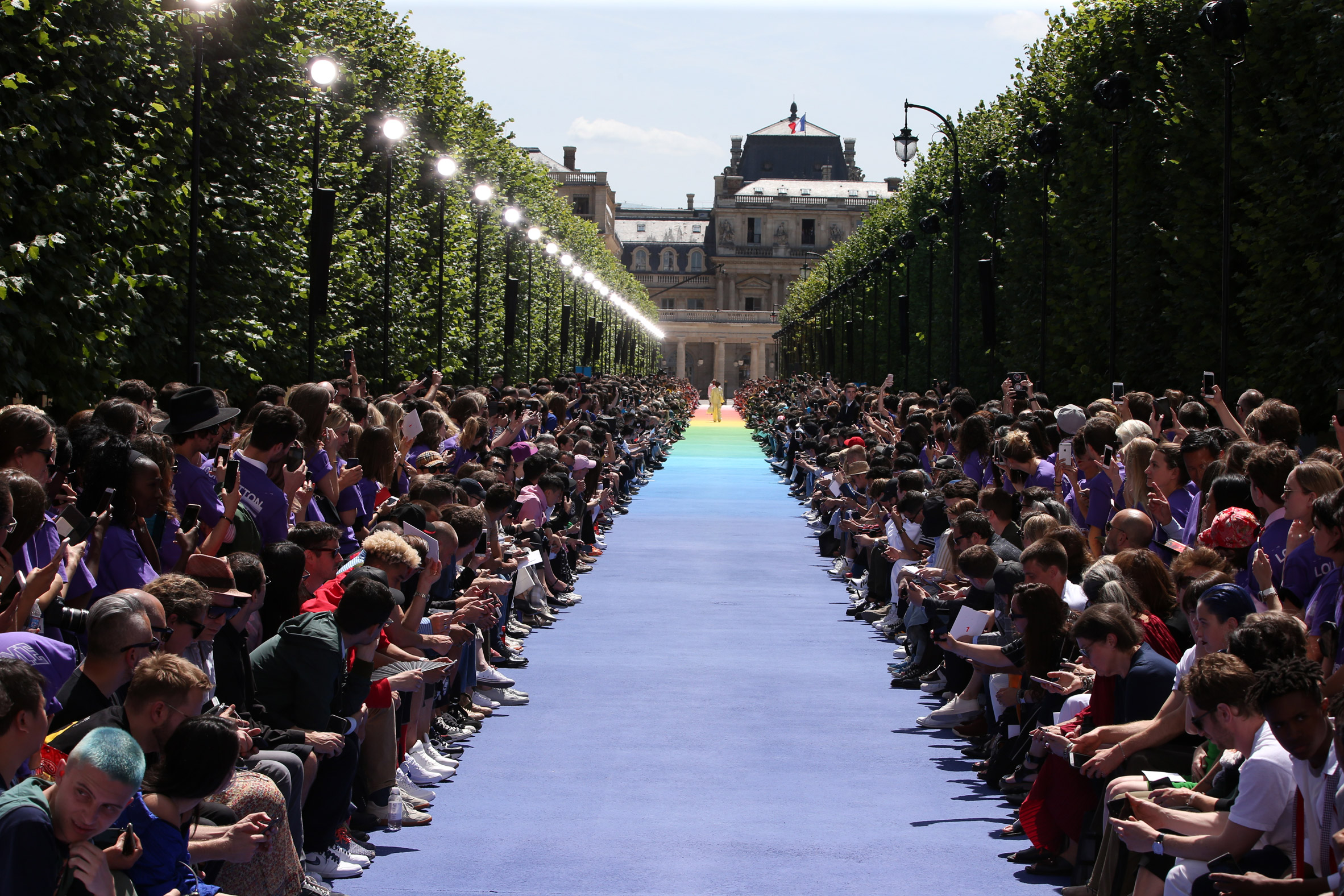This image captures a vibrant runway show set on a paved walkway leading towards a large, ornate building, resembling a castle. The walkway is bordered by tall hedges, lined with light poles—only the lights on the left side are illuminated. Hundreds of people, predominantly dressed in matching purple shirts, are assembled on either side of the walkway, some seated and others standing, many holding their phones aloft to capture the event. In the distance, a solitary figure clad in a yellow or cream suit walks towards the building, their features indiscernible due to the distance. The scene is bathed in daylight, under a pale light blue sky, adding to the grandeur of this special ceremony.